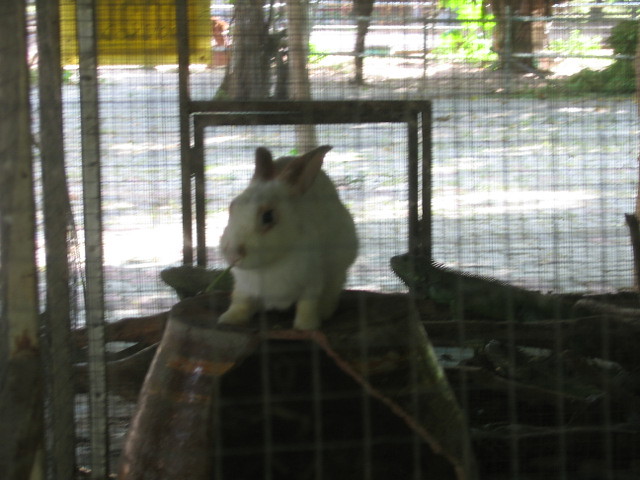This image features a white rabbit with a brown circle around one of its black eyes and dark brown accents on its ears. The rabbit is perched on a brown barrel, which is situated at the center of the image. Its setting appears to be a cage, crafted from wire or chicken wire, filled with various items including tools and stands that contribute to its busy appearance. To the right of the rabbit, there is a green iguana. The cage seems to be part of a zoo or an animal enclosure, as indicated by the presence of these exotic animals. In the background, you can see a walking path and perhaps the beginning of a tree, with a possible sign positioned in the top left corner, adding context to the outdoor environment. The ground inside the cage is a whitish-gray color, and the overall dimness and blur in the photo add a somewhat indistinct quality to the details.